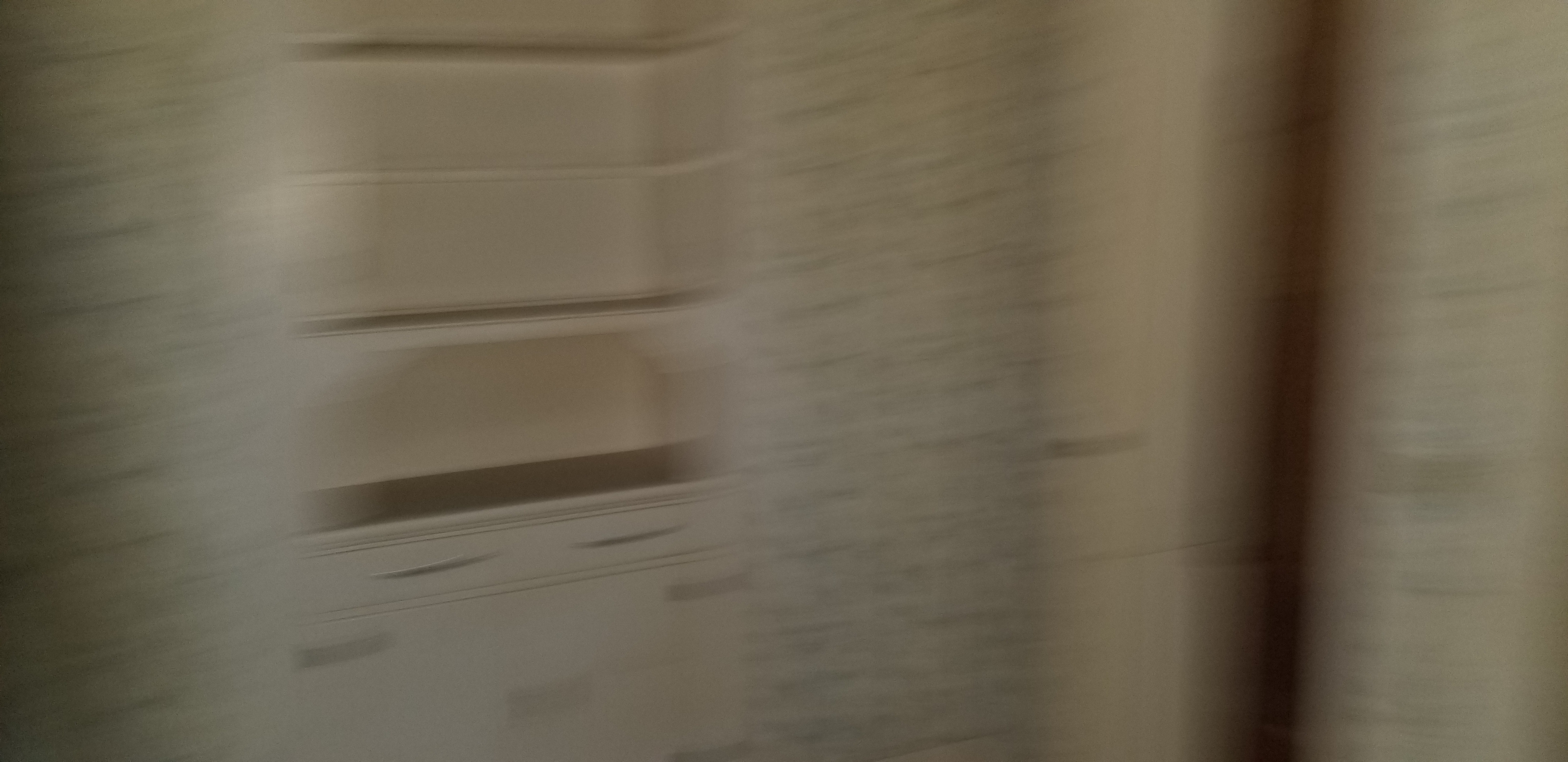A dark, grainy, and extremely blurry image shows the dimly-lit interior of a room, characterized by patterned wallpaper and a built-in shelf or cupboard inset into a wall. The structure, possibly featuring drawers and a cupboard, appears to be painted in a cream or off-white color. The yellowish tint suggests a poor lighting condition, potentially an overhead light that fails to illuminate the room adequately. The image is taken at a diagonal angle, with a noticeable corner post from floor to ceiling visible on the left wall and a possibly nearby doorway on the right-hand side. The scene includes light reflections that obscure finer details, making it difficult to distinguish specific patterns or contents of the room. Adjacent to this, a book with glossy reflections, dark writing, and tinged colors lies within the frame, suggesting it is old and has been exposed to smoke. The details of this book, such as potential drawings of a window, bed frame, and mattress, remain indistinct due to the image’s poor quality.